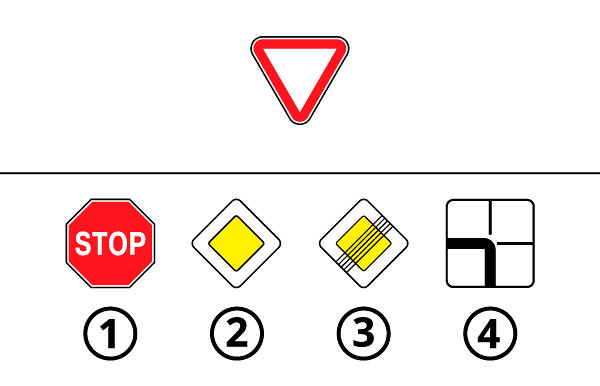The image showcases a collection of various traffic signs on a white background. At the top of the arrangement is an inverted triangle enclosed by a black outer border followed by a thick red inner border, with a white interior. This sign is blank without any text or symbols. Below this triangle, a straight black line horizontally bisects the image.

Beneath this line are four distinct traffic signs, each numbered for identification. 

1. **Sign Number 1:** This is a classic stop sign, characterized by its red octagonal shape and prominent white "STOP" lettering in the center.
2. **Sign Number 2:** Appearing as a diamond shape (a square turned 45 degrees), this sign features a thin black outer border, a thicker white inner border, and an additional black border framing a bright yellow center.
3. **Sign Number 3:** Identical in shape and borders to Sign Number 2, this sign is distinguished by five diagonal black lines crossing from one side to the other.
4. **Sign Number 4:** This is a square sign outlined in black, segmented by thick black lines extending from the top, right, bottom, and left edges, all converging at the center.